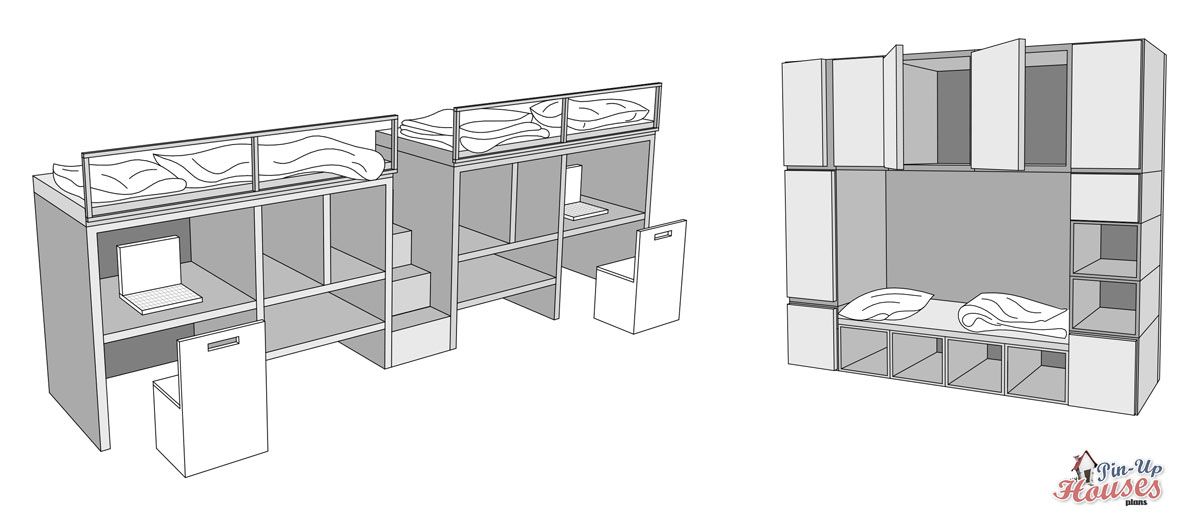This black and white schematic illustrates a multifunctional dorm-style living space designed by Pin-Up Houses. On the left side, there are two workstations, each equipped with a chair and a laptop, resembling college study areas. Above each workstation is a bunk bed complete with a pillow and blanket, accessible by a staircase located between the desks. Below and above the sleeping areas are locker-like cabinets and open shelves for storage. On the right side, another bed with similar shelving and cabinets is present. The image showcases a comprehensive guide to assemble this space-efficient furniture, suitable for both sleeping and working. The design emphasizes practicality and efficient use of space, ideal for dormitories or compact living environments.